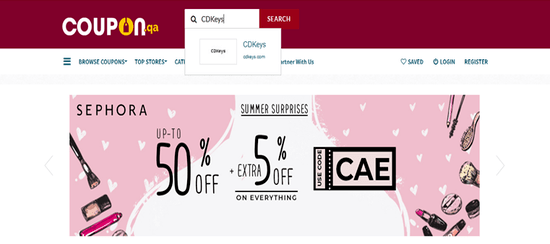Here is an organized and detailed descriptive caption based on the provided information:

---

At the head of the webpage titled "Rose," there's a prominent logo on the top left corner reading "coupon.QA." The letter "O" and the ".QA" are highlighted in orange, while the rest of the text "coupon" is displayed in white. Adjacent to this logo on the right side, a search box is positioned, featuring a red search button. Inside the search box, the placeholder text reads "see the keys," and this phrase also appears in the suggestion dropdown, both in blue font. The background of this suggestion page is white.

Beneath the header, a navigation bar showcases clickable text links in blue. Starting from the top left, the links read: "Browser," "Coupons," "Top Stores," "Categories." On the far top right, the options "Saved," "Login," and "Register" are also listed in blue. The entire background of the header is white.

In the center of the webpage is a featured coupon in a striking pink and white design. The coupon is adorned with illustrations of various makeup items, such as brushes and lipsticks. At the top of this section, bold text declares "Summer Surprises." On the top left corner of the coupon, the brand "Sephora" is noted in black text. The coupon promises "Up to 50% off plus an extra 5% on everything" with the use of the code "CAE."